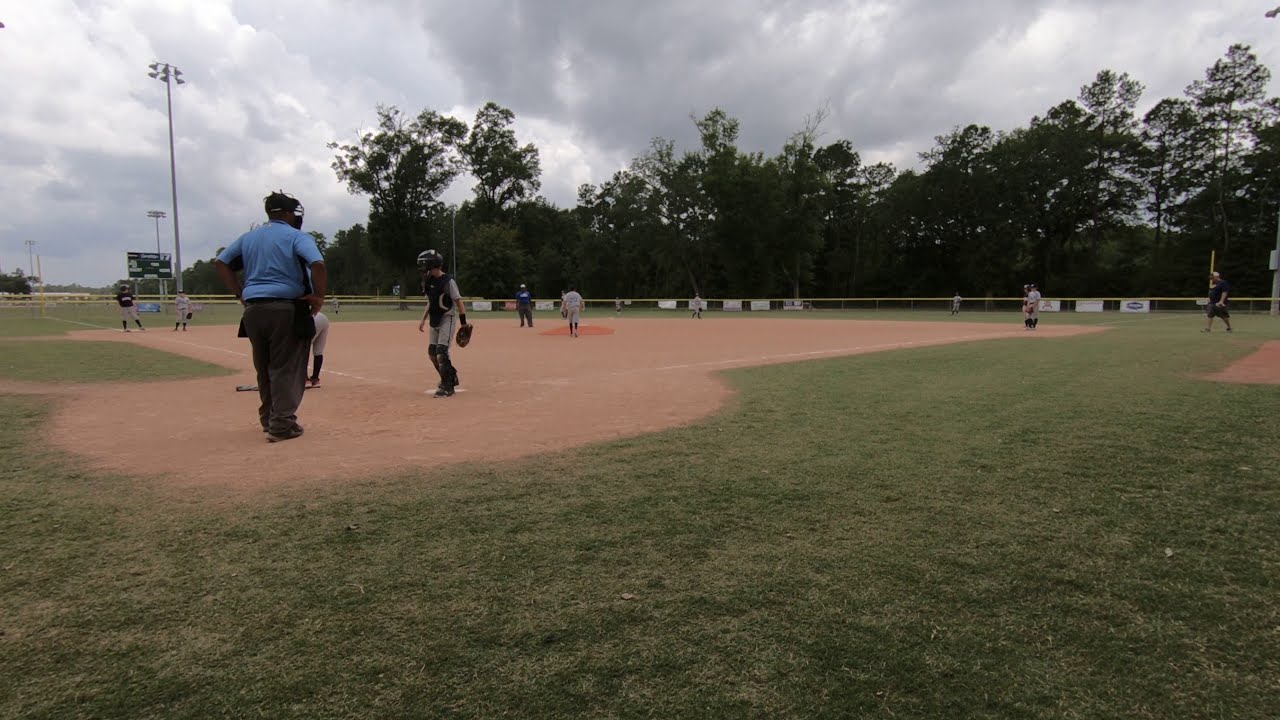The photograph captures an active baseball game on a lush green field, framed by a sky filled with dark and white clouds. Taken from behind the umpire, who is dressed in a blue shirt, brown pants, and a face mask, the image shows him standing behind home plate. A catcher in a pale sky blue shirt and black pants is also present, with his face mask down and hands on his hips. In front of the catcher, a young player with a baseball helmet and catcher's glove is ready for action. 

The infield is distinctively pink, contrasting with the green outfield. Players are positioned on first, second, and third bases, with a runner on third. A bat lies on the ground near home base, suggesting recent activity. In the far background, large stadium lights and a scoreboard can be seen. Tall green trees line the perimeter of the field, adding to the natural setting. Beyond the outfield, tall light poles and additional players in the distance further illustrate the bustling scene. The cloudy sky hints at impending weather, adding a dramatic backdrop to the game in progress.